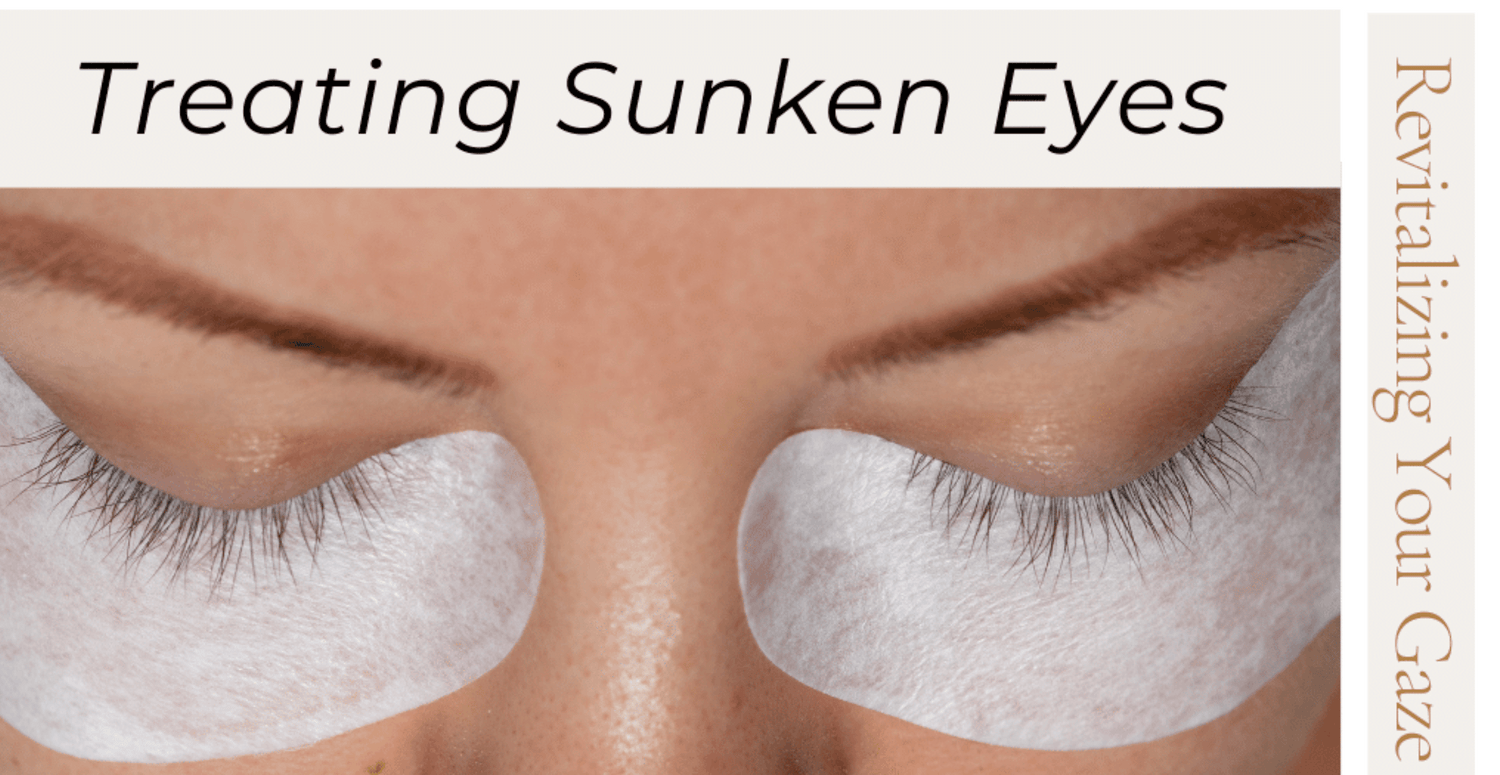### Treating Sunken Eyes

This image advertises a treatment for sunken eyes. At the top, in black font, the title "Treating Sunken Eyes" is prominently displayed. Along the right side, a tagline reads "Revitalizing Your Gaze."

The image zooms in on the eyes of a white woman whose face is partially visible. Her eyes are closed, and thin, brown eyebrows arch above. The eyebrows appear to be meticulously drawn, giving a precise look. Below her closed eyes, protective white patches made of cotton are evident, enhancing the impression that she is undergoing a treatment. These patches curve in a creasing shape beneath her black eyelashes. The woman's nose is visible between the patches, revealing fine pores and casting a slight shadow on each side. The overall focus is on her eye region, emphasizing the detailed care being taken to address the appearance of sunken eyes. The mouth is not visible in this tightly cropped image.